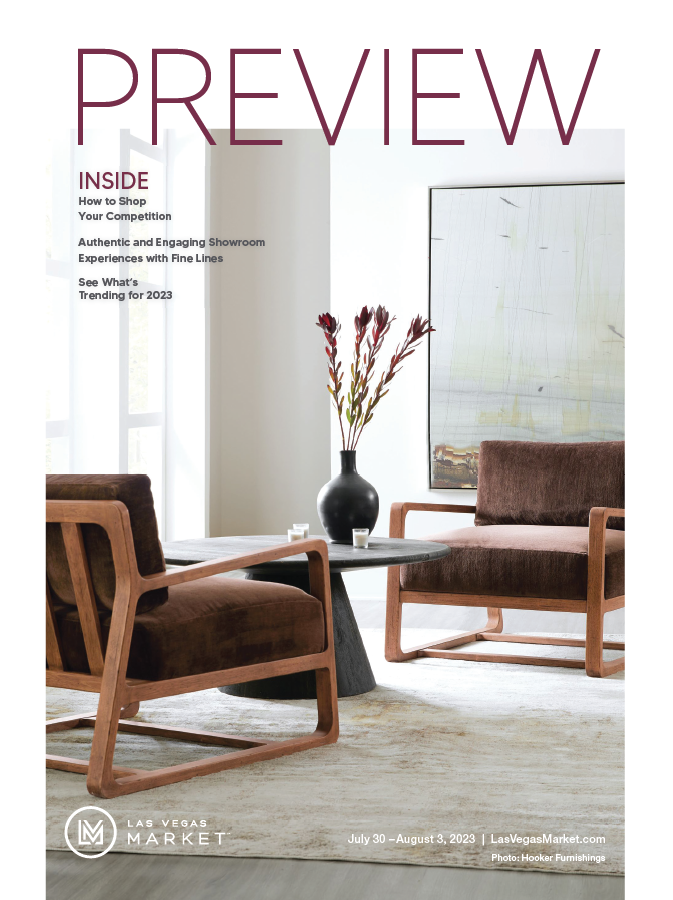The cover of the Las Vegas Market magazine for July through August 2023 features a modern furniture setup in a sunlit showroom, characterized by stark white walls and a light-colored carpet. Prominently displayed at the top in large red letters is the title “PREVIEW,” suggesting either the magazine’s name or a sneak peek of its contents. Below that, headings include “INSIDE: How to Shop Your Competition” and “Authentic and Engaging Showroom Experiences with Fine Lines,” followed by “See What's Trending for 2023.”

The room’s arrangement includes two wooden-framed chairs with thick brown cushions, positioned opposite each other. Between them stands a small, round mushroom-shaped table with a flared pedestal. Adorning the table is a black vase holding four red flowers and three white votive candles in glass containers. An abstract painting with brown hues at the bottom hangs on the wall, adding to the room's contemporary aesthetic. At the bottom of the cover, the logo reads “LAS VEGAS MARKET,” with details noting the event dates, July 30th through August 3rd, 2023, and the website LasVegasMarket.com. Additionally, the photograph credit reads “PHOTO HOOKER FURNISHINGS.”